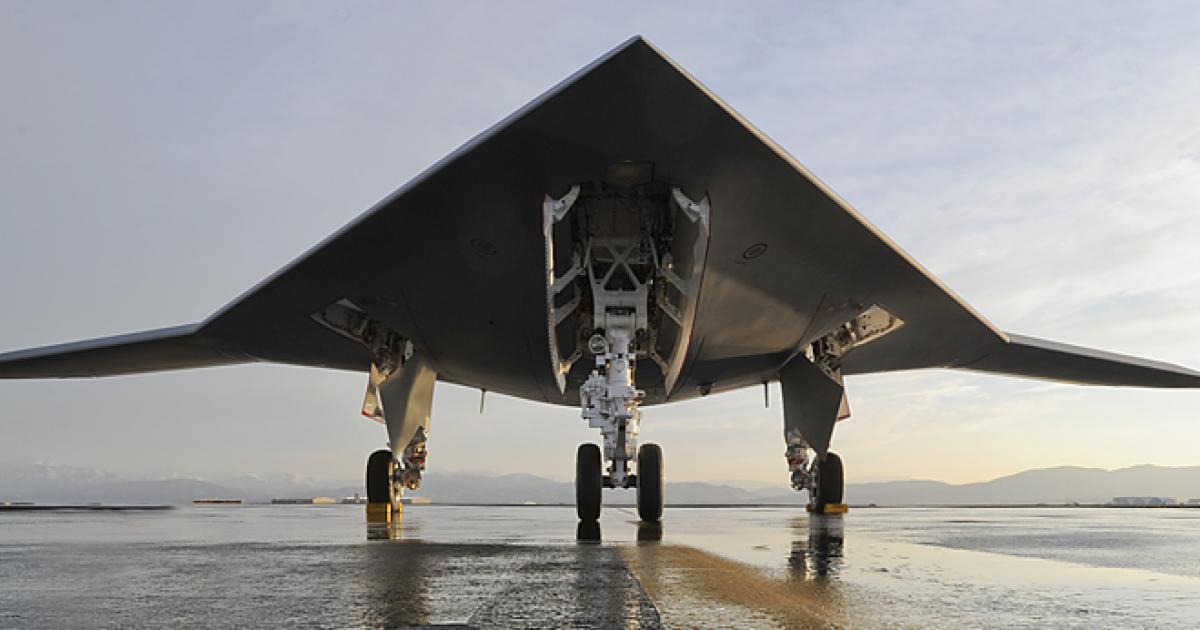In this image, we see what appears to be an F-35 stealth bomber situated on a wet taxiway, reflecting a recent rain. The aircraft exhibits a distinctive deltoid shape with a narrow, pointed V-shaped nose and short, stubby wings. This sleek, triangular craft is supported by three landing gear sets: one under the nose and one beneath each wing. Although no markings, flags, or people are visible, the aircraft's detailed design commands attention. The background reveals mountains in the distance under a light blue sky interspersed with clouds, while additional buildings can be spotted along the horizon, adding to the expansive, open setting.